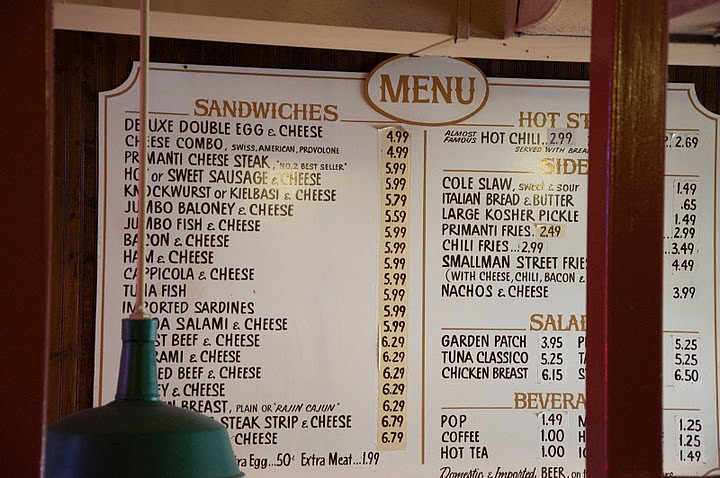This photograph captures a detailed view inside a vintage-style deli restaurant. Dominating the image is a large, wall-mounted menu, broader than it is tall, positioned centrally for easy visibility. At the upper center, a circle sign prominently labeled "Menu" marks the top of the board. On the left side, under the gold-lettered "Sandwiches" heading, a list of various sandwiches is presented in black lettering. Offerings include options such as Deluxe Double Egg and Cheese, Cheese Combo, and Jumbo Fish and Cheese. Each sandwich price is marked on removable sticky paper, ranging from $4.99 to $6.79.

Obstructing a portion of the menu on the right side is a red pole, while on the left, a green lamp suspended from a thick tube covers some of the letters. Despite these obstructions, the right side of the menu is categorized with items such as "Hot Sandwiches," "Sides," "Salads," and "Beverages." Side options include Coleslaw, Italian Bread and Butter, and Large Kosher Pickles. Salads listed are the Garden Patch, Tuna Salad, and Classic Chicken Breast. Beverage choices feature Pop, Midwestern-style Coffee, and Hot Tea.

Overall, the menu exudes an old-timey charm, characteristic of a classic sandwich joint or deli, where patrons can easily peruse their choices while waiting in line.